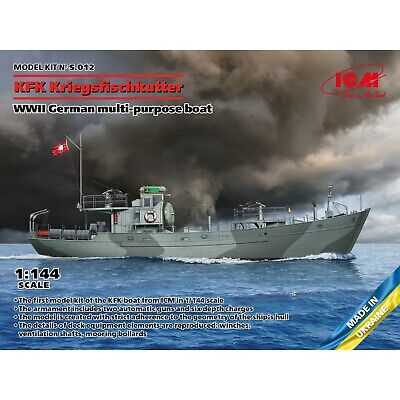This detailed photographic advertisement showcases a model ship kit, labeled as KFK Kriegsfischer Kutter, a World War II German multipurpose boat. The model is identified as Kit No. NS012 and is to a 1:144 scale. The name "KFK Kriegsfischer Kutter WWII German multipurpose boat" is prominently displayed in black lettering below the title "Model Kit" in red letters on the top left-hand corner. The brand "ICM" appears in red text on the top right-hand corner, indicating the manufacturer. The model box cover features a detailed illustration of the boat, which is styled similarly to a PT boat and rendered in gunmetal gray.

Central in the image, the boat is depicted sailing through crystal blue water, trailing dark gray smoke from smaller smokestacks on its deck into what was once a clear, blue sky. The boat's wheelhouse features a hint of green detailing, and at the ship's rear, a tall post flies a red flag with a white center. Additional notable details include a black and light red life preserver attached to the passenger container on the vessel.

The bottom left corner of the image contains additional specifications in black font, while the bottom right corner displays a yellow diagonal banner with white text reading "Made in Ukraine." This banner also includes the Ukrainian flag, emphasizing the model's origins.